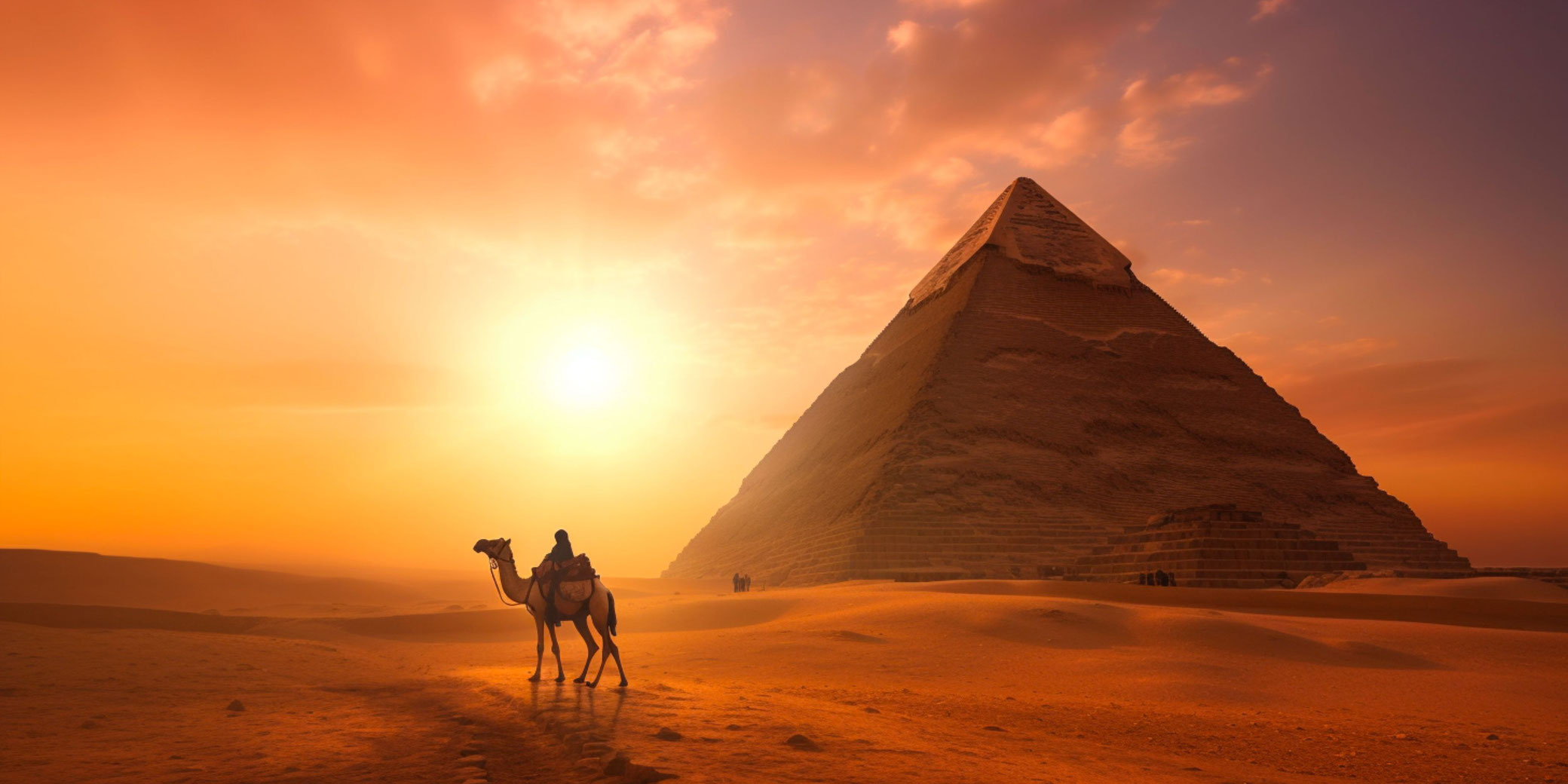The image beautifully captures an ancient pyramid in the desert at sunset. The sky, predominantly orange-yellow with patches of blue and scattered clouds, features the ball of the sun positioned left of center. To the right of the glowing sun stands the pyramid, bathed in warm hues of brown and orange reflecting the twilight. The structure displays two visible sides, one facing right and the other left, with a cap area at its top. In the lower portion of the image, the sands are tinted orange, shaped into various small dunes by the wind. A lone silhouette of a rider on a camel is seen to the left of the pyramid, traversing the desert landscape. The overall scene, possibly derived from a video game illustration, is imbued with a surreal, almost enhanced color palette, adding to the mystique and beauty of this timeless desert view.